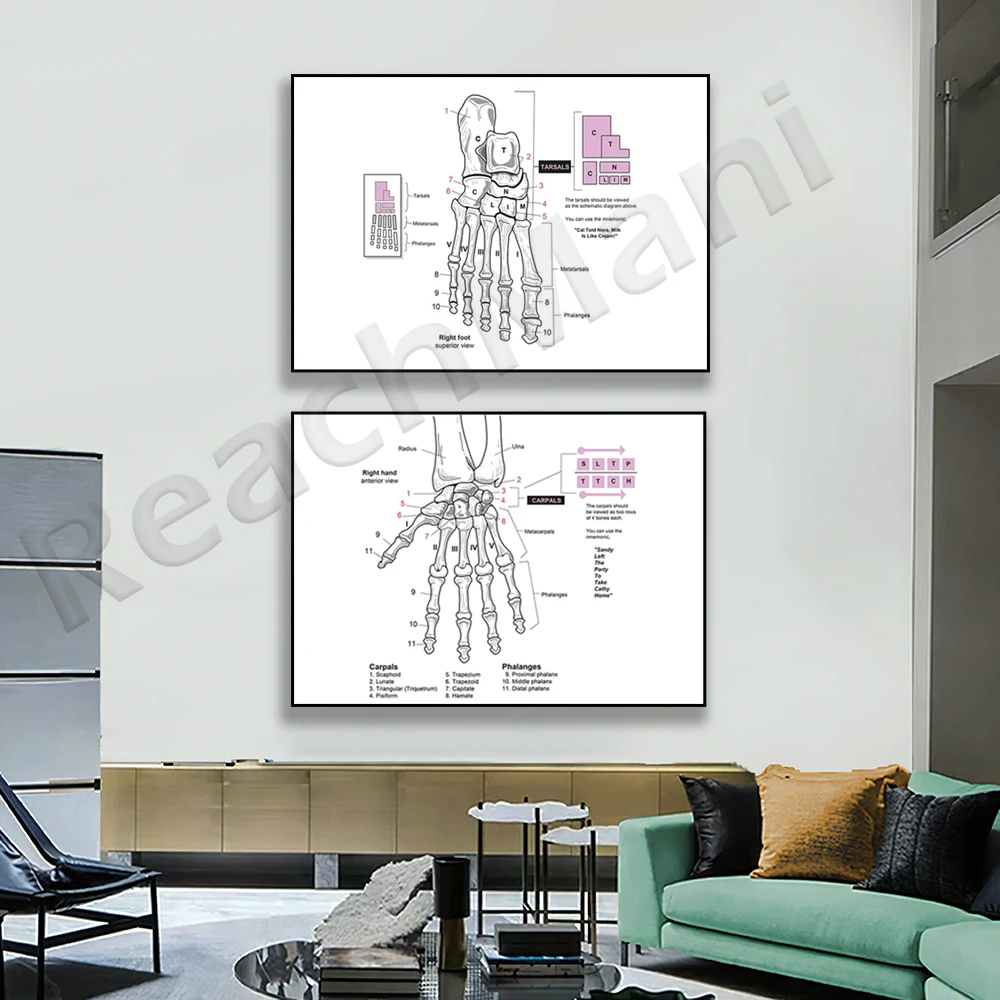This photograph portrays a spacious room, likely a doctor's office, characterized by medical diagrams and comfortable seating areas. Dominating the white wall are two large diagrams—one depicting the skeletal structure of a foot at the top and the other showing the reverse side of a hand at the bottom, complete with labels identifying various joints and digits. A watermark reading "Reach Money, M-A-N-I," or possibly "Reach Ilani," spans diagonally across the image, making it somewhat challenging to decipher. 

The interior features a green couch adorned with black and orange pillows on the right side, accompanied by a central coffee table cluttered with several books. Adjacent to the couch is a black, deep-seated reclining chair. On the left-hand side, amidst light brown storage cabinets and a tall silver file cabinet, tiles add a distinctive touch to the decor. The background includes a gray divider screen and a large window, contributing to the room's open and airy atmosphere.